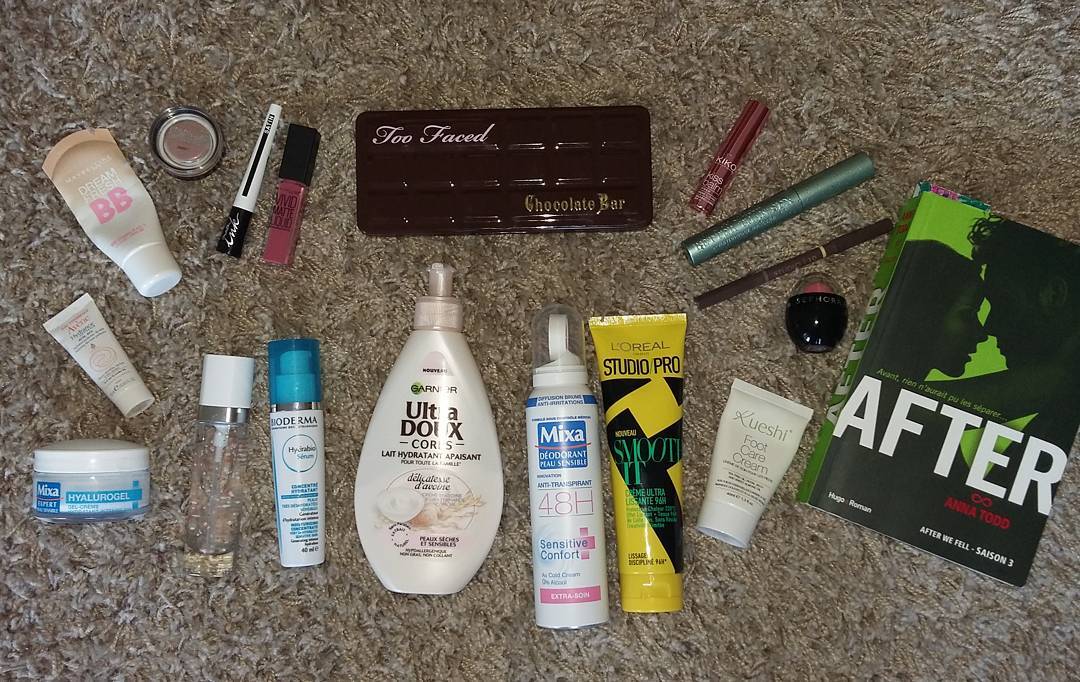This photograph captures an assortment of cosmetic products meticulously arranged on a carpet beside a book. Among the items, there is a Two Feast chocolate bar adding a sweet touch to the display. The beauty products include bottles of mascara, a brown eyeliner pencil, and a vibrant yellow tube of L'Oreal Studio Pro with the label "Smooth It." There is also Mike's deodorant, which promises "48 Hours Sensitive Comfort," and an Ultra Dough hydrant aspirant for added skincare. Not to be overlooked is the Maybelline Dream Fresh BB cream, perfect for a light, fresh-faced look. Positioned on the far right, the book titled "After" features a cover illustration of two people embracing, contributing to the intimate and personal atmosphere of the scene. This detailed collection highlights a variety of beauty essentials and a leisurely reading choice, all laid out on a cozy carpet backdrop.